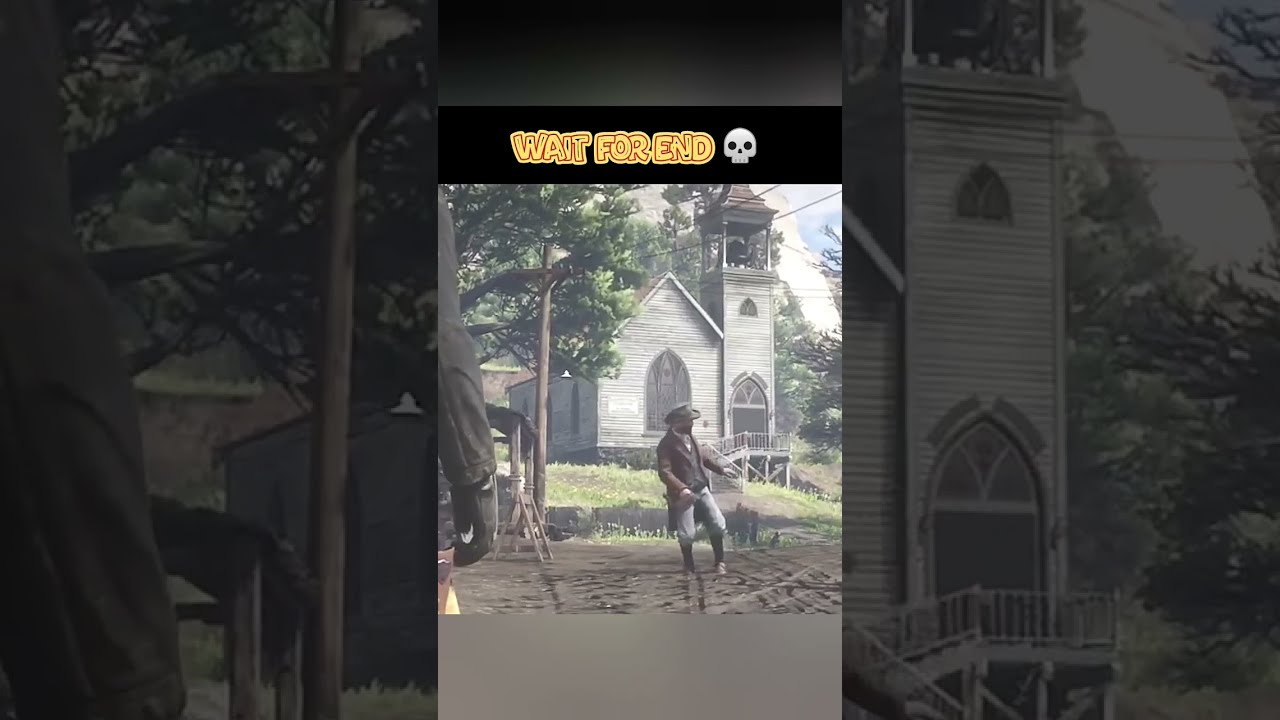The image is a horizontal rectangle divided into three panels that combine to form a single cohesive visual narrative. The left and right panels darken the overall image and are identical, each depicting the right side of an old white church building with a bell tower, a deciduous tree set against the background of more trees, and faintly visible tree limbs across the top. A man’s arm appears partially in the foreground, cut off at the bottom and left edge.

The center panel, which appears imposed over the left and right panels, offers a clearer, lighter, and more distant view of the same scene. Here, a man, possibly a character from a video game, is seen walking towards the viewer, wearing a brown cowboy hat, a brown long-sleeved jacket, and knickers-like pants. He is standing on dry ground, which appears muddy in places, with grass and more trees partially visible near the church. The man looks back over his left shoulder, his hand more clearly visible than in the left panel.

A distinct feature of this central panel is the text "wait for end" in yellow letters accompanied by a skull icon located towards the top, framed by a black border. The same image details continue towards the right panel where the darkened church’s right side and steps leading up to it are visible, along with more tree scenery in the background.